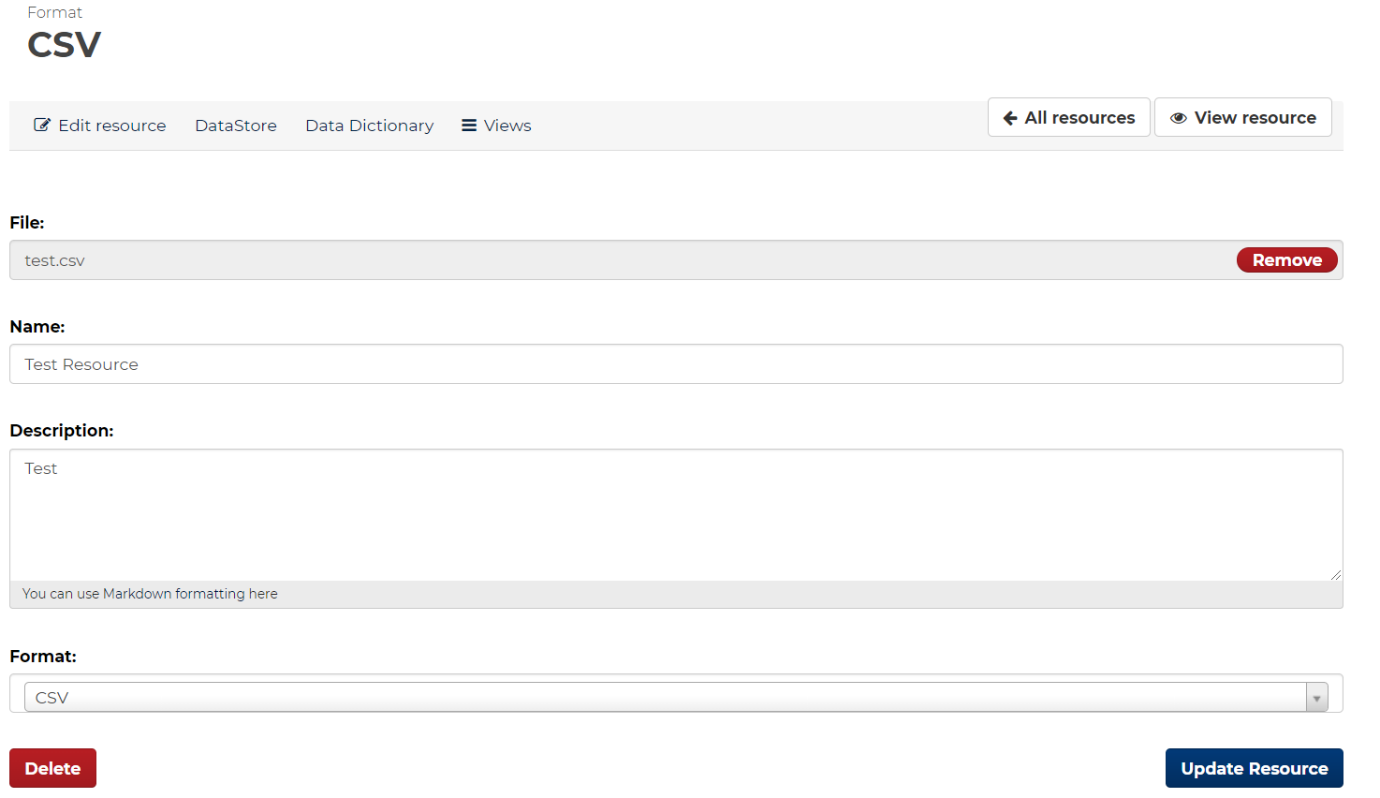The image depicts a structured form against a white background. At the top left corner, the text "Format: CSV" is displayed in black. Below this heading, various navigational tabs are lined up vertically on the left side, including "Edit Resource," "Datastore," "Data Dictionary," and "Views."

On the top right corner, there are two white buttons, "All Resources" and "View Resource," both labeled in black text.

The left portion of the form begins with a section labeled "File," in which the inserted file is named "test.csv." Adjacent to this file name on the right side is a white button labeled "Remove" in black text. Directly below the file section is a "Name" field filled with "test resource."

Continuing down is a "Description" field containing the text "test," with an empty space still in white. Just beneath the description, there's a note indicating that "You can use Markdown formatting here."

At the very bottom of the form, the text "Format" appears, with a drop-down menu selected to "CSV." Two buttons are positioned at the bottom: a red "Delete" button on the left side and a blue "Update Resource" button on the right, both inscribed with white text.